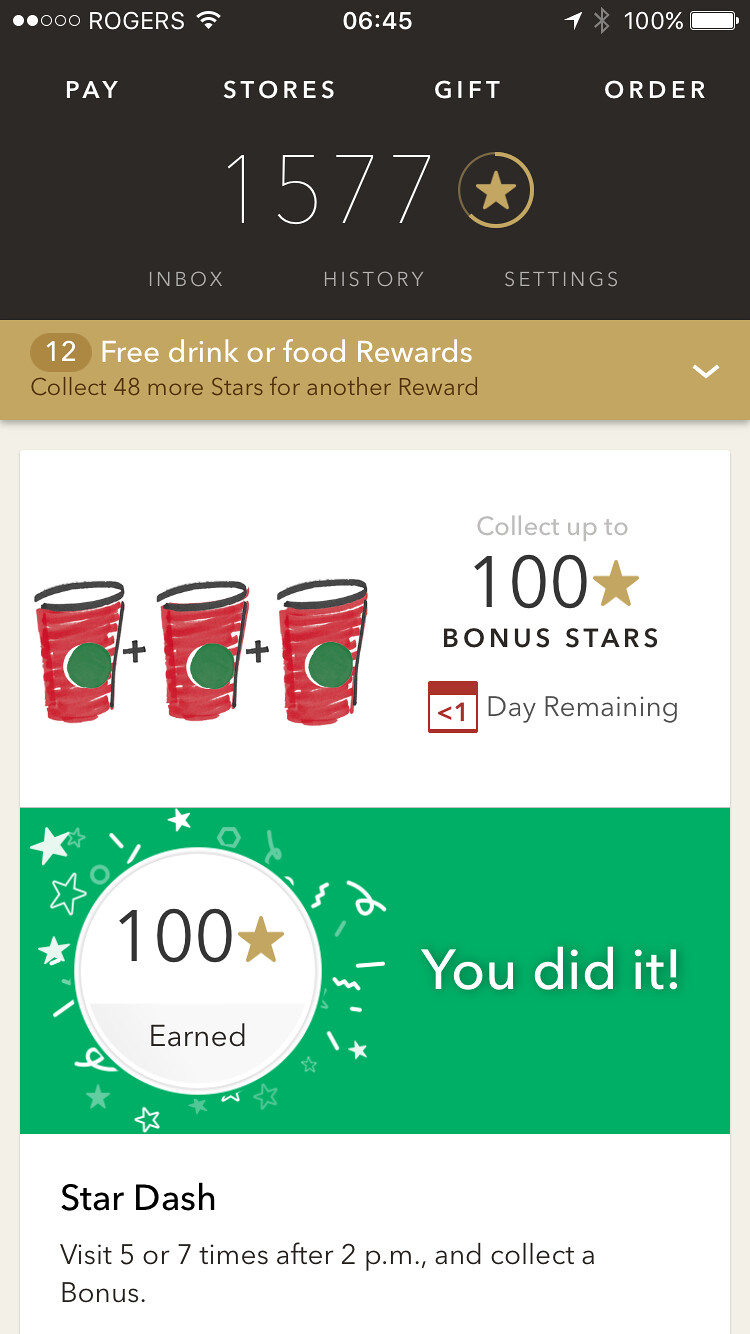This is a detailed screenshot of an iOS phone, specifically displaying the Starbucks app. At the very top, the status bar indicates full Wi-Fi signal beside the carrier name "Rogers," the time "6:45" without specifying AM or PM, full battery, and an active location tracker icon. Below this, the app's navigation bar includes options labeled "Pay," "Stores," "Gift," and "Order." Prominently displayed in a large font is the number "1577" next to a circular star icon, representing the user's accumulated Starbucks points. Directly beneath this, the app displays tabs labeled "Inbox," "History," and "Settings."

Further down, in a highlighted bar, it shows "12 free drink or food rewards," along with a message stating "Collect 48 more stars for another reward." Another promotional section features illustrations of three Starbucks cups and advises users to "Collect up to 100 bonus stars" with "less than one day remaining," accompanied by a green progress bar confirming "100 stars earned" and celebrating with the phrase "You did it" and confetti graphics. Finally, a panel at the bottom details a "Star Dash" promotion that encourages visiting five to seven times after 2 p.m. to collect a bonus.